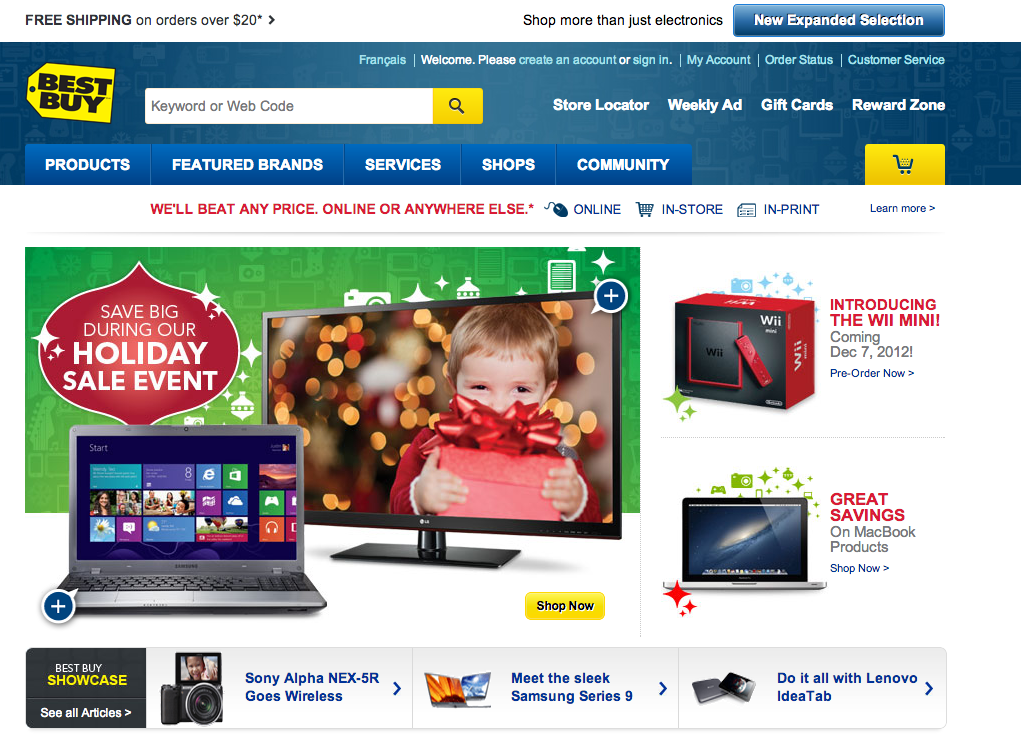This image depicts the homepage of the Best Buy website, featuring a well-organized and visually appealing layout. 

At the top left corner, the iconic Best Buy logo is prominently displayed in black text against a vibrant yellow background. To its right lies a search bar, while further to the right, a yellow square with a magnifying glass icon serves as the search button. Adjacent to the search bar are four categories in white text: Store Locator, Weekly Ad, Gift Cards, and Reward Zone.

Above these categories, options in light blue text offer links for Create an Account or Sign In, My Account, Order Status, and Customer Service. Directly below, a navigation bar in dark blue with white text features five tabs: Products, Featured Brands, Services, Shops, and Community. Another yellow square with a shopping cart icon is situated to the right of these tabs.

Beneath the navigation bar, bold dark red text declares, "We will beat any price online or anywhere else," accompanied by options for Online, In-Store, and In-Print. An eye-catching advertisement below this statement reads, "Save Big During Our Holiday Sale Event," set against a red ornament-like background. The advertisement features images of a laptop and a TV.

To the right of the advertisement is a section introducing 'WeMint,' followed by a segment highlighting "Great Savings on MacBook products," complete with a "Shop Now" icon. At the bottom of the page, three gray tabs with blue writing provide additional navigation options. In the bottom left corner, a black square marked with “Best Buy” features the term “Showcase” in yellow text.